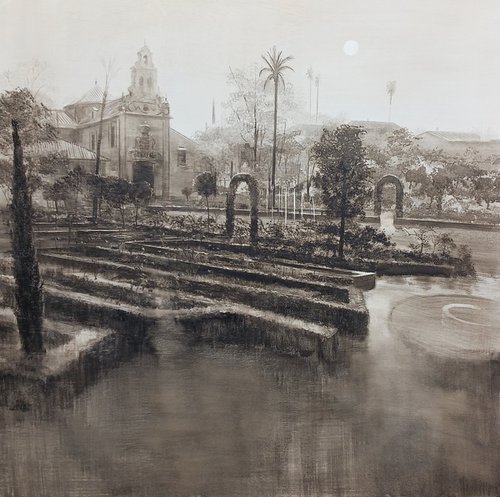The black-and-white image, which has a vintage feel reminiscent of a pencil drawing or early photograph, depicts a sunlit scene with intricate details. Dominating the foreground on the left side is a meticulously manicured garden with maze-like patterns and cement enclosures, likely housing a variety of plants. At the middle right of the image, tall palm trees reach upwards, their presence mirrored by more palms in the background. Towards the back left of the image stands a prominent building, resembling a cathedral or church, which extends from the middle to the far left, distinguished by its grayish-brown tones. The sky, shaded in grays and whites, features a bright sun near the center-right. Adding to the tranquil ambiance, a round fountain rests at the middle right, hinting at the presence of water in the garden's layout.